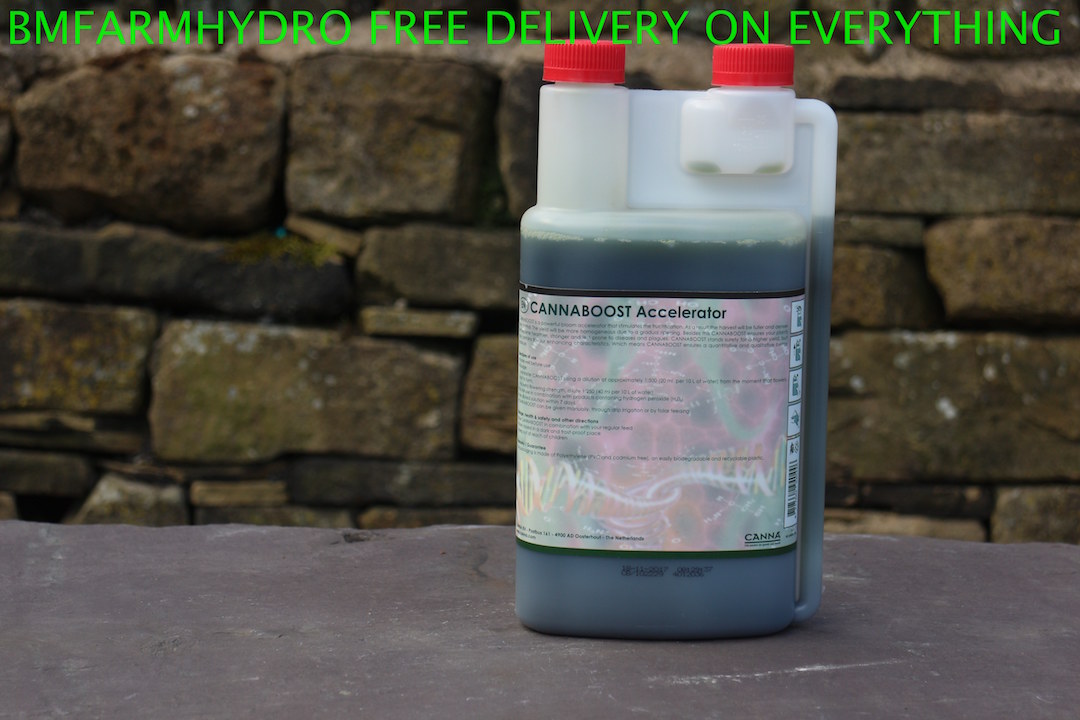This color landscape photograph prominently features a large white plastic container filled with a dark blue-gray liquid, identified by the label as "Canna Boost Accelerator." The container, which has two red caps on the top—one on the left for the main reservoir and one on the right for a smaller connected reservoir—is positioned slightly to the right of center, occupying a significant portion of the image from top to bottom. The bottle rests on a smooth slate gray surface, while the backdrop features a rough, brown-red brick wall that adds depth due to the applied depth of field. Above the container, bright green text reads "BM Farm Hydro Free Delivery on Everything," suggesting a farm supply context. The label on the container is detailed but with text too small to discern beyond the main headline. This photograph is an example of photographic representational realism, capturing the subject with clarity and detail.